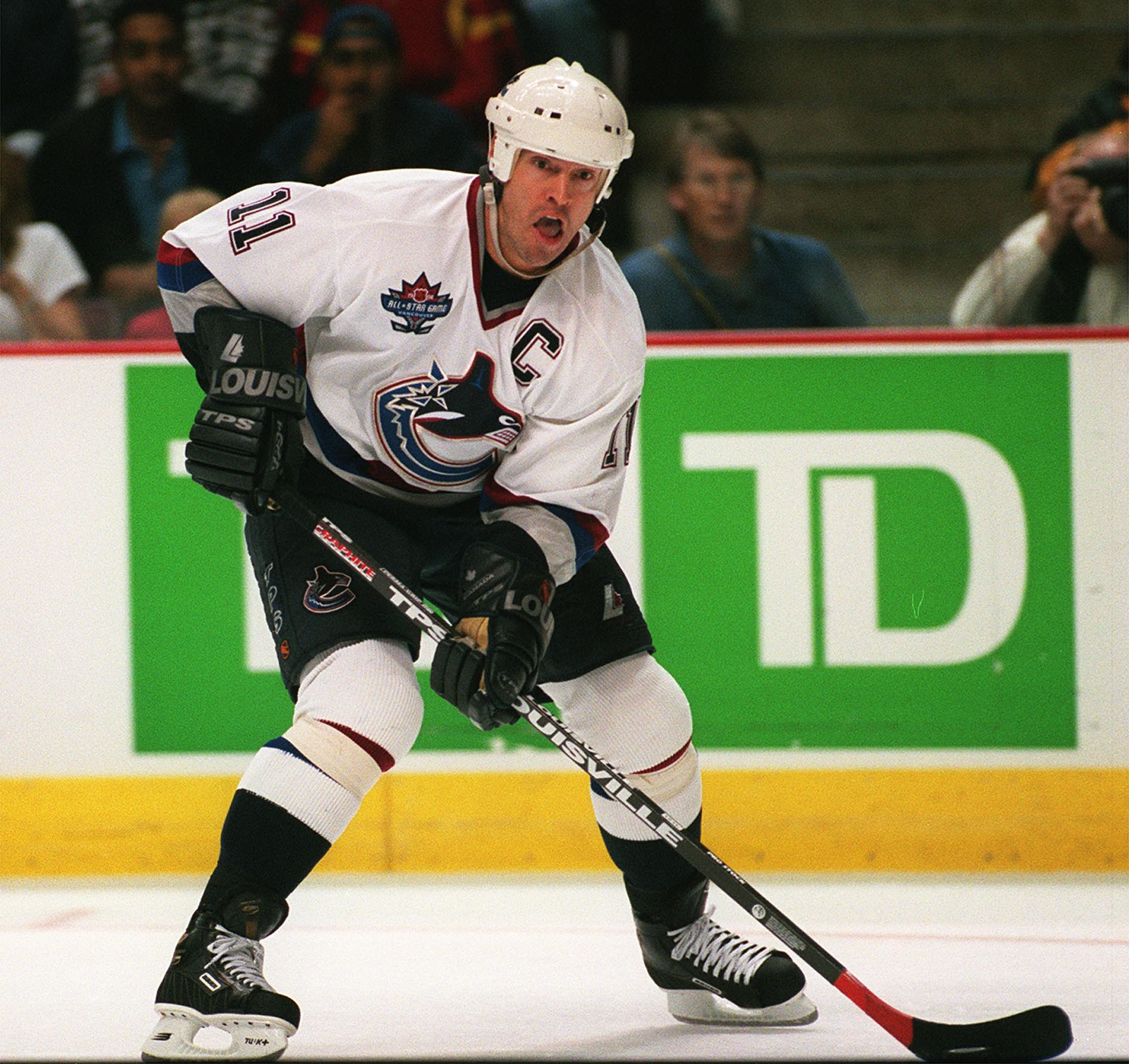In this image, we see a detailed and dramatic photograph of a hockey player on the ice. The player is wearing black skates and is equipped with white knee protection pads, thick black gloves which prominently feature the word “Louisville” and the acronym “TPS.” He also has black shorts, a white jersey with the number 11 on his shoulders, and a white helmet for protection. The player is gripping a black hockey stick that includes a red border outline at the bottom and white letters near the end, and features a bit of red tape just before the curve of the stick.

The center of his white jersey displays a distinctive emblem depicting a shark breaking out of a letter "C," accompanied by a maple leaf and the words "All-Star" at the top left, and another letter "C" on the top right. His expression is one of shock or bewilderment, with his mouth slightly open, as if reacting to something unexpected.

In the background, we observe a blurry crowd of about six to eight spectators in the stands. The rink's protective wall below them displays a green square advertisement featuring the white letters “TD,” with a yellow strip running along the bottom of the wall. This combination of focused and background details captures the intensity and atmosphere of the hockey rink perfectly.